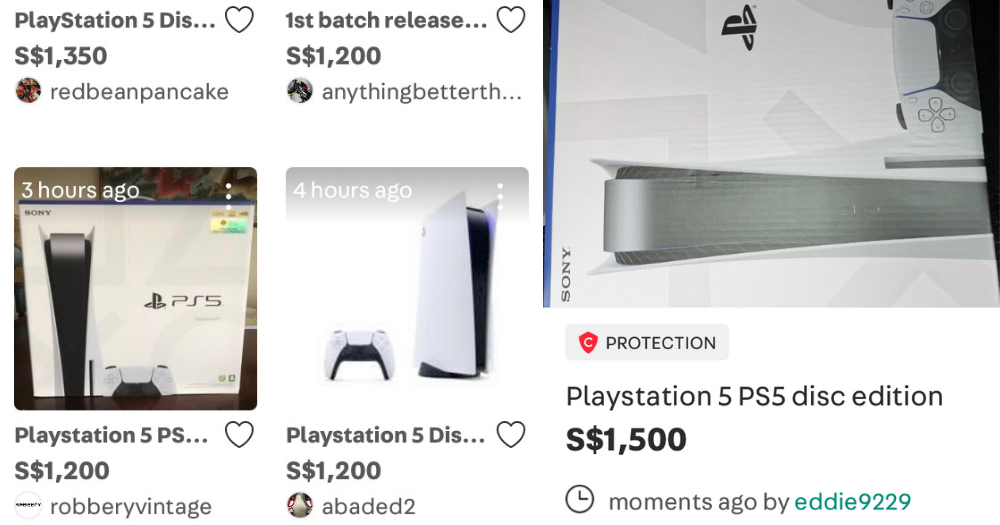The image has a plain white background and features several listings for PlayStation 5 consoles. At the top left, there is a heading that says "PlayStation 5 DIS..." accompanied by a heart icon and a price of $1,350. Below this, there is a small profile picture with the username "red bean pancake."

To the right of this, there is another listing that reads "First batch release..." with a heart icon and a price of $1,200. Underneath, there's a profile picture with the username "anything better th..." This listing is noted as being posted three hours ago and shows an image of a PlayStation 5 box.

Below this, another listing states "PlayStation 5 PS..." with a heart icon and a price of $1,200, accompanied by a profile picture with the username "robbery vintage."

The final listing is timestamped four hours ago and features an image of a PlayStation 5 box alongside a video game controller. The caption reads "PlayStation 5 DIS..." with a heart icon and a price of $1,200.